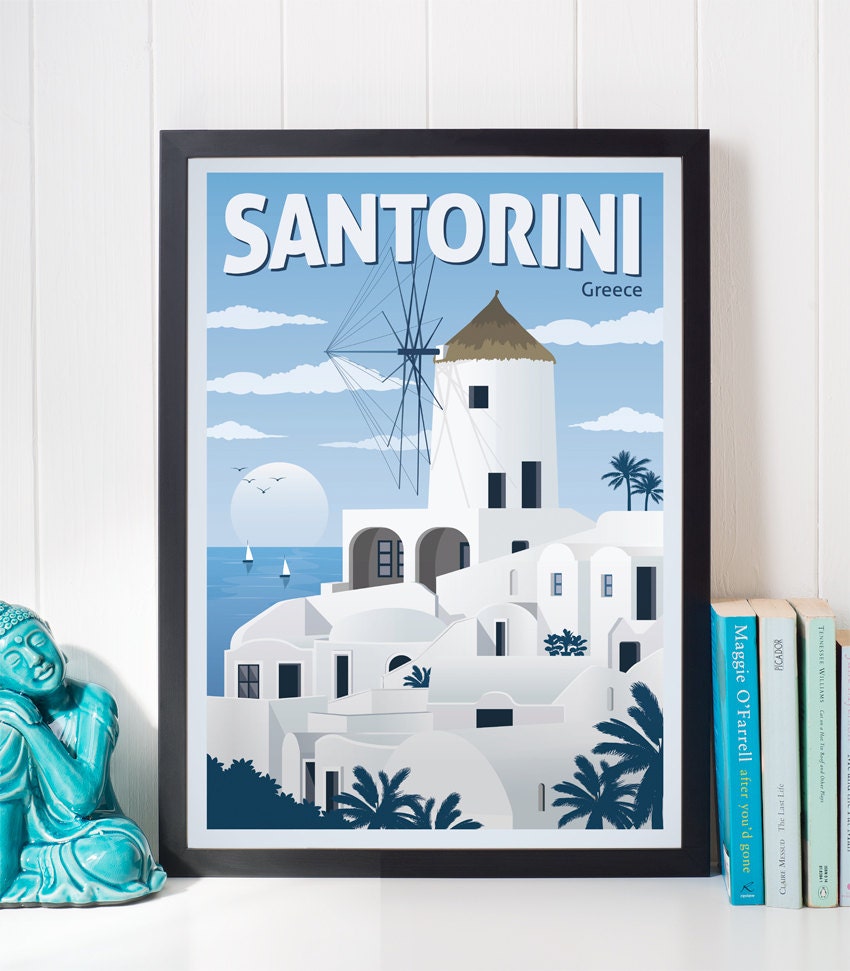This image depicts a stock photo setup featuring a serene and organized shelf scene. At the center of the composition is a framed Santorini, Greece poster with a black border. The poster showcases an idyllic, computer-illustrated coastal landscape of white buildings with brown thatched roofs, intricate windows, and doorways, intermingled with lush green palm trees. The background displays a blue sky adorned with fluffy white clouds and a bright white sun or moon, accompanied by a few birds and sailboats over the tranquil water. 

To the left of the framed poster is a contemplative teal ceramic Thai Buddha statue, sitting with one leg crossed and one knee bent, head resting on its arms in a meditative pose. Slight white fading adds a delicate texture to the Buddha figure. On the right side, four books of assorted colors are neatly lined up. Prominently visible among them is "After You’d Gone" by Maggie O’Farrell, alongside volumes in shades of white, teal, robin’s egg blue, and another less discernable book. The scene is beautifully set against a plain white wood panel wall, with the white surface of the shelf or table completing the minimalist, calming aesthetic.